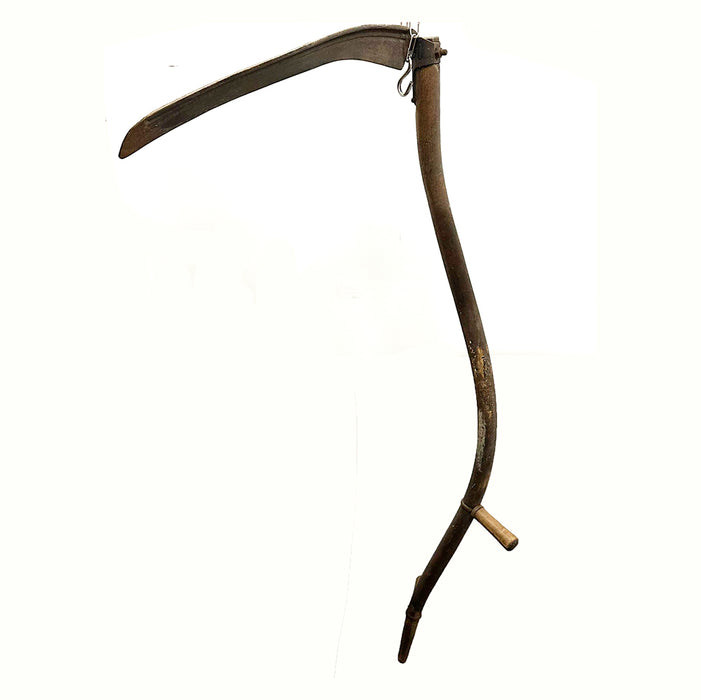This image is a color photograph of an antique farming scythe set against a white background. The scythe features a long, slightly curved wooden handle that appears weathered and damaged in some areas. Attached to this handle is a smaller handhold intended for additional bracing while in use. The blade of the scythe is long, angled downward, and pointed to the left. It shows signs of aging, with visible browning and rust at the tip. Overall, the scythe has an aged and worn appearance, reflecting its historical use in culling grain or wheat on a farm.